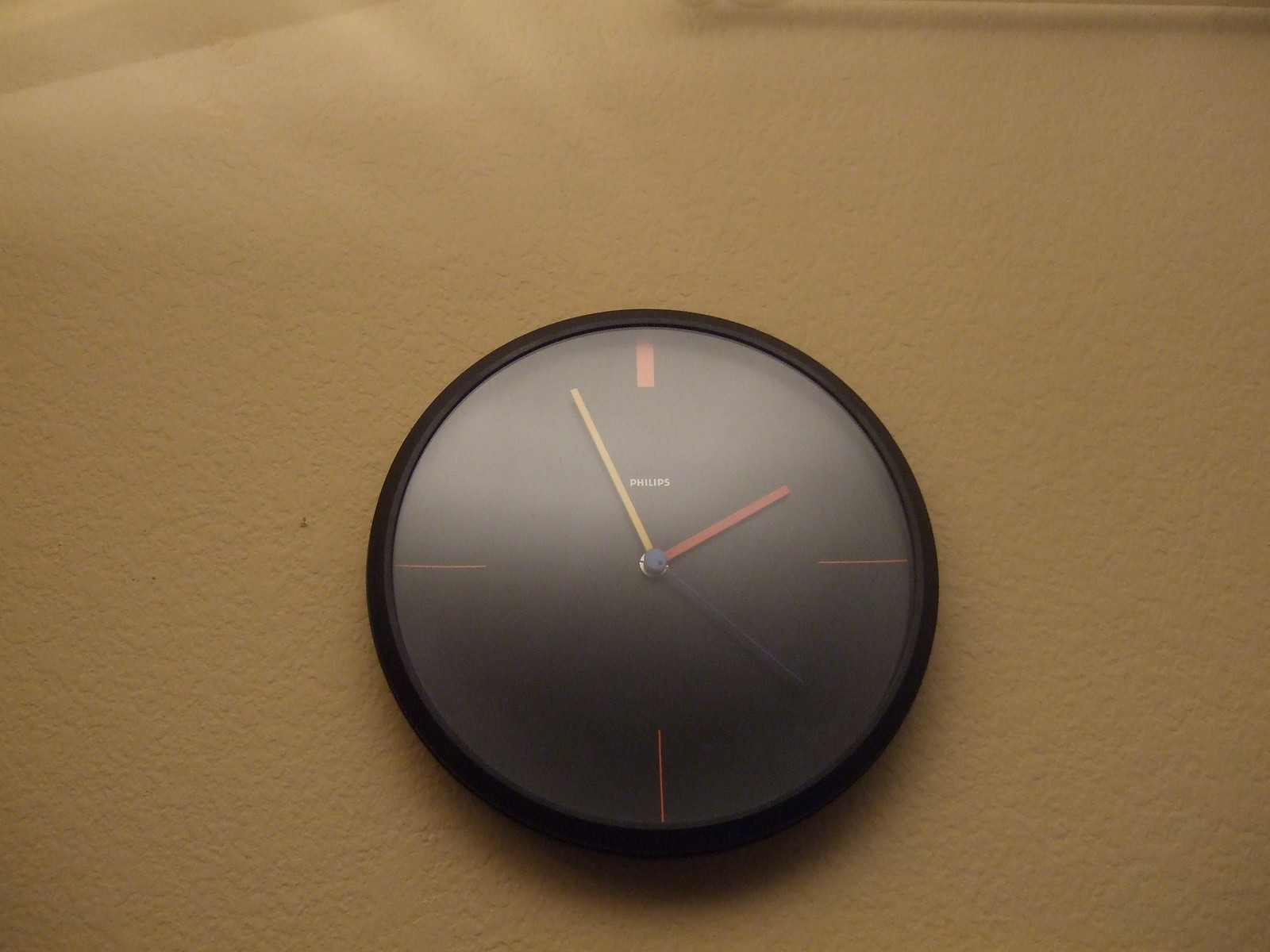This detailed photograph showcases a modern Philips wall clock set against a beige background. The clock features a sleek design with a black rim and a black-and-silver face. Notably absent are traditional hour numbers; instead, the 12, 3, 6, and 9 positions are marked by vertical notches, with the 12 o'clock mark being the thickest. The brand name "PHILIPS" is prominently displayed just below the 12 o'clock position. The clock's hands are distinctively colored: the hour hand is black, the minute hand is reddish, and the second hand is yellowish. The clock appears to indicate a time around 1:55, with the second hand approaching the 20-second mark. The image focuses solely on this contemporary clock, highlighting its unique and minimalist design.